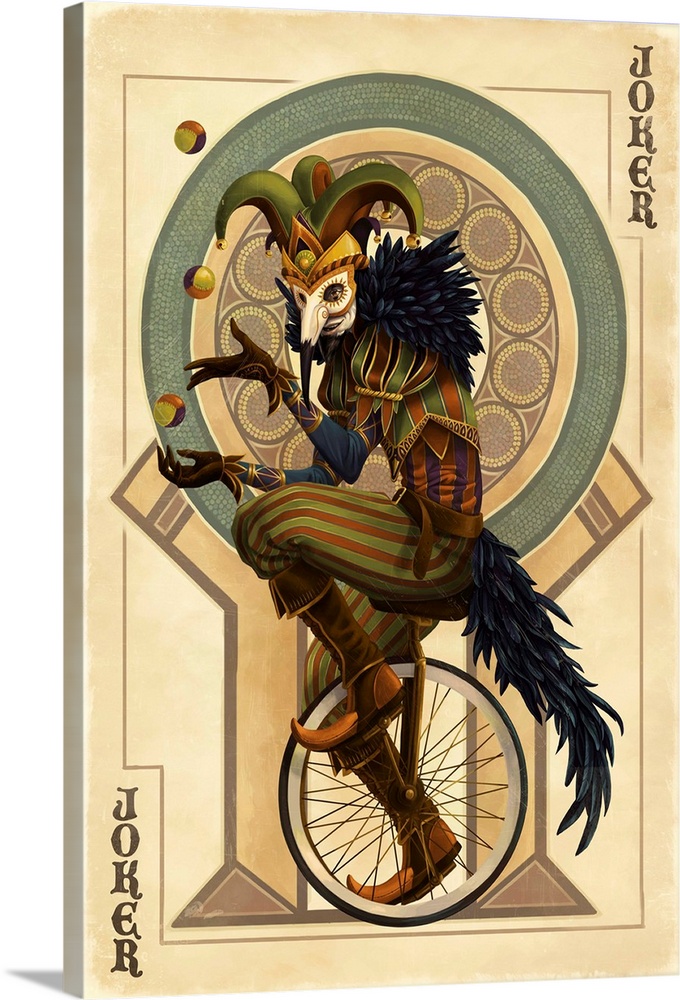This image portrays an old-style Joker playing card printed on aged, tan-beige paper. The card prominently features the word "Joker" written in an old English script in both the top right and bottom left corners. Dominating the card is a whimsical figure of a jester on a black unicycle. The jester, clad in an elaborate costume, sports a hat with three sides ending in bells and a mask reminiscent of a Plague Doctor's mask, conferring a long nose and an air of mystery.

The jester’s outfit is vividly detailed with orange and green striped pants, green and orange striped vest, and extravagant green boots with curled toes. His shoulders are adorned with puffy elements made of black feathers accented with blue, which also constitute a cape trailing behind him. The jester is seen skillfully juggling three multicolored balls in gold, orange, and black. Additionally, there is a design element behind him that resembles a large circle with smaller circles within it, adding to the lively and fantastical ambiance of the artwork.